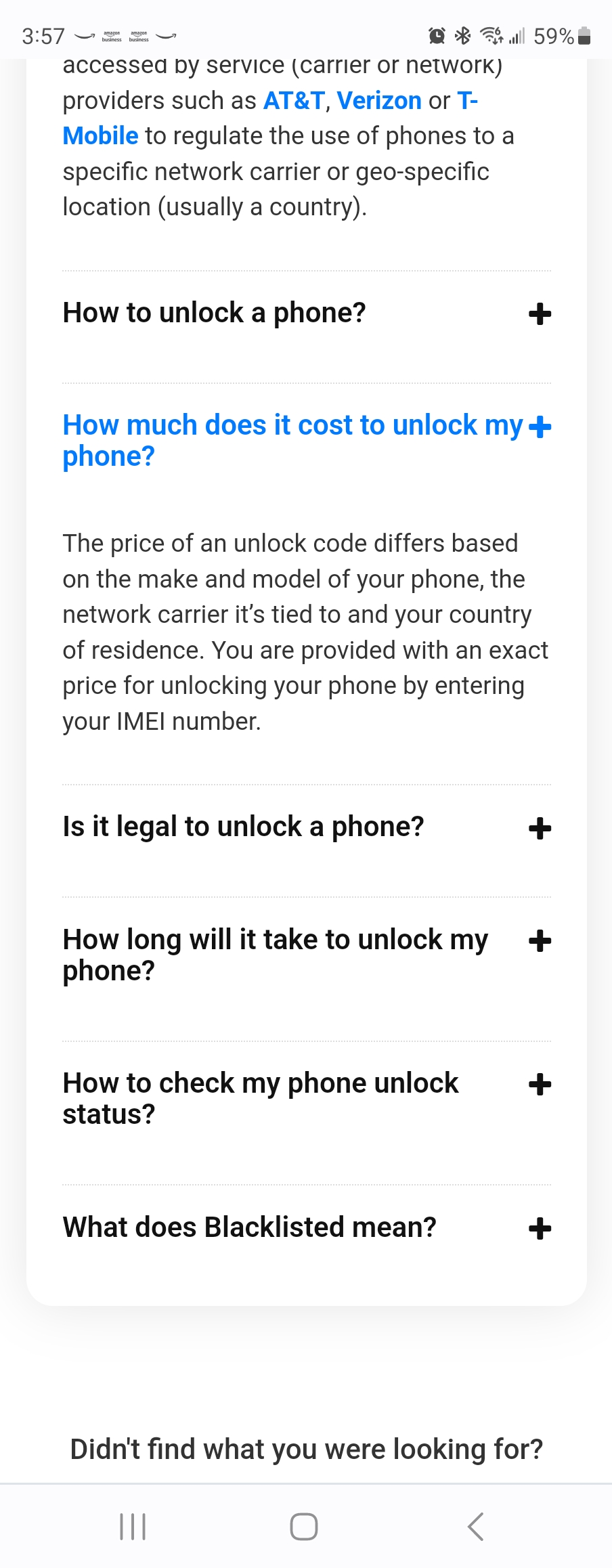The image shows an FAQ page being viewed on a mobile phone at 3:57 pm. The phone screen indicates that it has an active alarm set, Bluetooth is enabled, and it is connected to a 4G network with three out of five signal bars. The battery is at 59%. 

The FAQ page contains a large amount of text. The first visible portion of text is partially cut off but mentions access by server, carrier, or network provider like AT&T, Verizon, or T-Mobile to regulate the usage of phones by network, carrier, or geographical location, usually by country.

A heading with a plus sign, indicating it can be expanded, reads "How to unlock a phone." Following that, there's an already expanded menu item in blue text stating, "How much does it cost to unlock my phone?" The content under this expanded item explains that the cost of an unlock code varies based on the phone's make and model, its network carrier, and the user's country of residence. The exact price for unlocking a phone can be determined by entering the phone's IMEI number.

There are four other menu items in bold black text, each with a plus sign next to them indicating they can be expanded. These items are:
1. "Is it illegal to unlock a phone?"
2. "How long will it take to unlock my phone?"
3. "How to check my phone's unlock status?"
4. "What does blacklisted mean?"

Below the list of questions, outside the white content box, a partial phrase "Didn't find what you're looking for?" is visible, followed by a cut-off section. Light gray lines separate each header or menu item.

At the bottom of the screen, the mobile interface displays navigation buttons: three vertical lines, a rounded square, and a back arrow (less than sign).